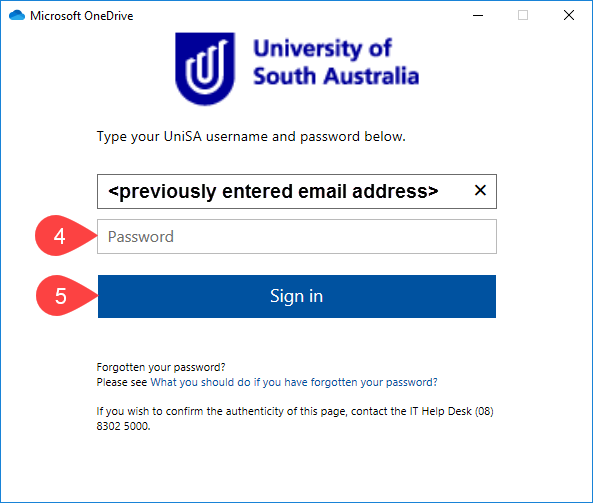The image displays a screenshot of a login webpage for the University of South Australia’s Microsoft OneDrive account. The page has a clean, white background. At the top left corner, there’s a "Microsoft OneDrive" label next to the OneDrive icon, which is a cloud with shades of blue and dark blue. Centrally positioned at the top is the "University of South Australia" text, written in blue, accompanied by the university's logo on the left - a blue emblem featuring two interlocking white "U"s.

Below the main header, a black text prompt instructs users to "Type your Unesa username and password below." Beneath this, there are input fields for the username (with placeholder text displaying a previously entered email address) and the password, respectively. To the left of the username input field, a red pointer labeled "4" is visible. Directly below the password field is a blue "Sign in" button with white text, accompanied by another red pointer labeled "5."

At the bottom of the page, there's a note stating: "Forgotten your password? Please see what you should do if you have forgotten your password. If you wish to confirm the authenticity of this page, contact the IT Help Desk at 0883025000."